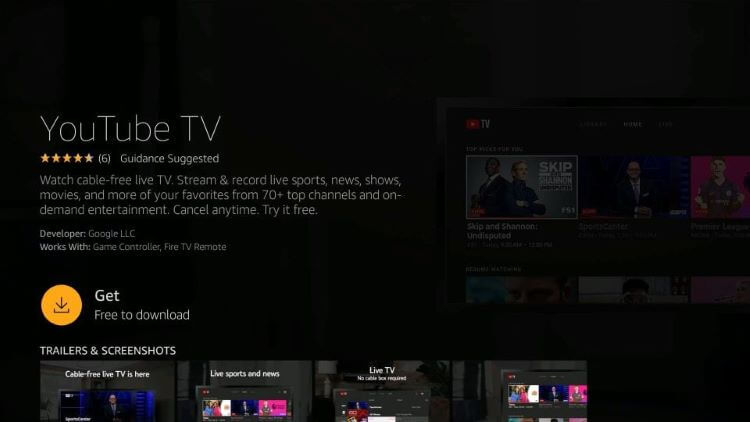The image showcases the landing page for downloading the YouTube TV app on an Amazon Fire TV device. The page features a predominantly black background with key information prominently displayed. At the top, the YouTube TV logo is visible, alongside a four-star rating and a "Guidance Suggested" label. The text promotes YouTube TV's offerings, highlighting the ability to watch live TV without cable, including live sports, news, shows, movies, and more from over 70 top channels and on-demand entertainment. It also mentions the convenience of canceling at any time and a free trial offer. Below this, the developer is identified as Google LLC, and there is a note that the app is compatible with game controllers and the Fire TV remote, confirming its use on Amazon Fire devices.

An orange button labeled "Get" is shown for downloading the app for free. The section titled "Trailers and Screenshots" appears below, with dark images representing various TV show examples. These images are somewhat difficult to discern due to their low brightness.